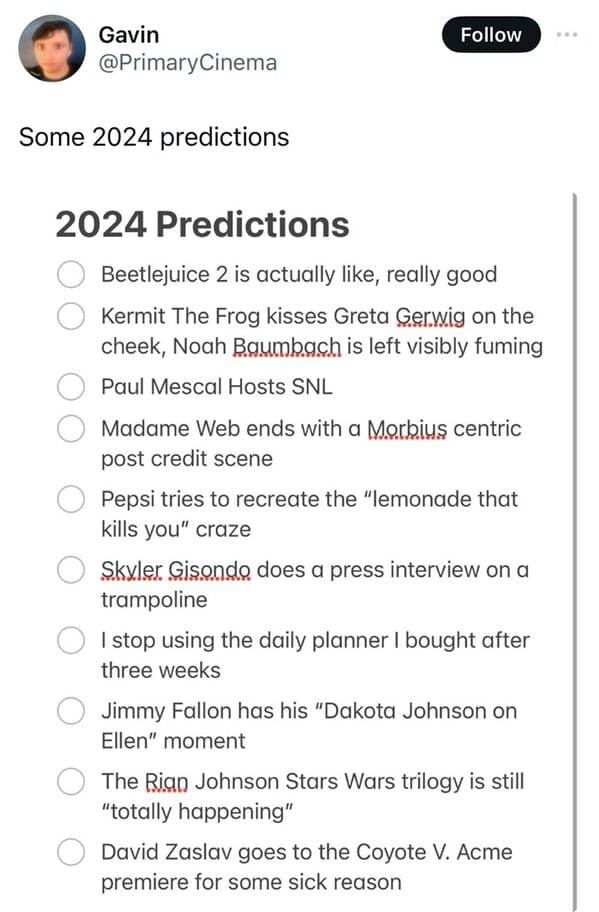In front of a minimalist, white background with black text, a vivid image encapsulates a series of witty and surreal predictions for 2024. In the center, Kermit the Frog is seen giving a gentle kiss on the cheek to Greta Gerwig, while a visibly fuming Noah Baumbach looks on. To the right, Paul Mescal steps in to host an SNL segment, as Madame Webb concludes with a dark, melancholic post-credit scene. Meanwhile, Pepsi attempts to revive the controversial 'lemonade that kills you' trend. Skyler Gisondo conducts an animated press interview while energetically bouncing on a trampoline. Further in the background, a comedic element is added with a mention of someone abandoning their daily planner after just three weeks. On another note, Jimmy Fallon experiences his own 'Dakota Johnson on Ellen' moment. The caption humorously assures that the Rian Johnson Star Wars trilogy is 'still totally happening.' Adding to the unexpected twists, David Zaslav makes an inexplicable appearance at the 'Coyote Walk' premiere of an Acme event. Interspersing the predictions is a gray circle with a white center. Some names are underlined in red due to spellcheck not recognizing them, adding an additional layer of intrigue to the scene.